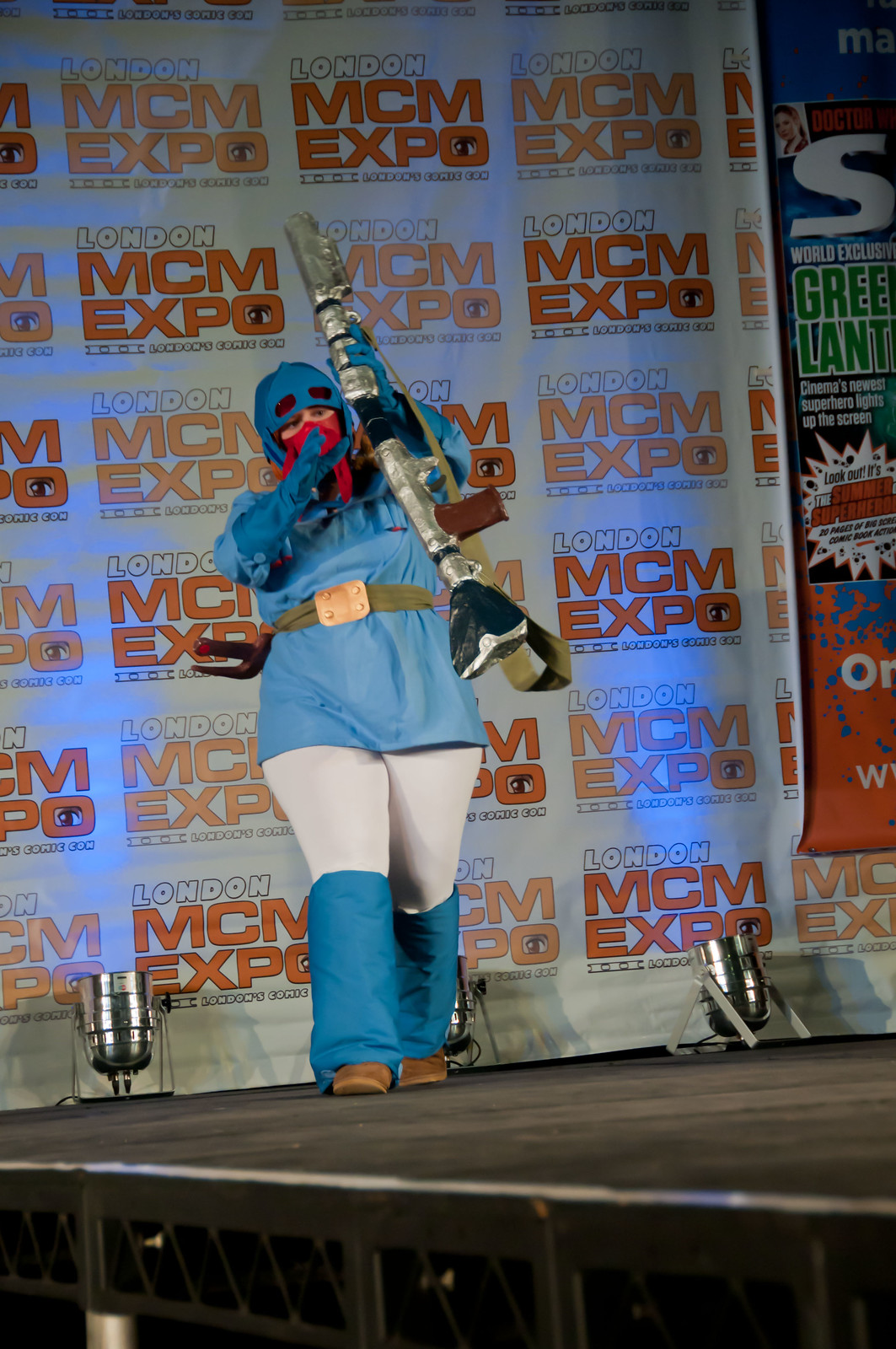In this detailed photograph taken at the London MCM Expo, a person is featured in the center of a stage under multiple lights, suggesting it is an indoor event. The backdrop reveals the text "London MCM Expo," confirming the cosplay setting. The individual is wearing a striking superhero-like costume, comprising white and blue pants, a long-sleeve blue shirt, blue gloves, and blue boots. They accessorize with a green belt, featuring a copper buckle around their waist, and a red bandana covering their mouth. A blue cap with holes for vision is also part of their disguise. The subject is holding a large, silver rifle, characterized by a handle and magazine, which they appear to be showcasing or possibly twirling. Additional objects such as stage equipment and lights are visible, contributing to the vibrant scene with multiple colors including silver, black, gray, white, blue, red, orange, and green.